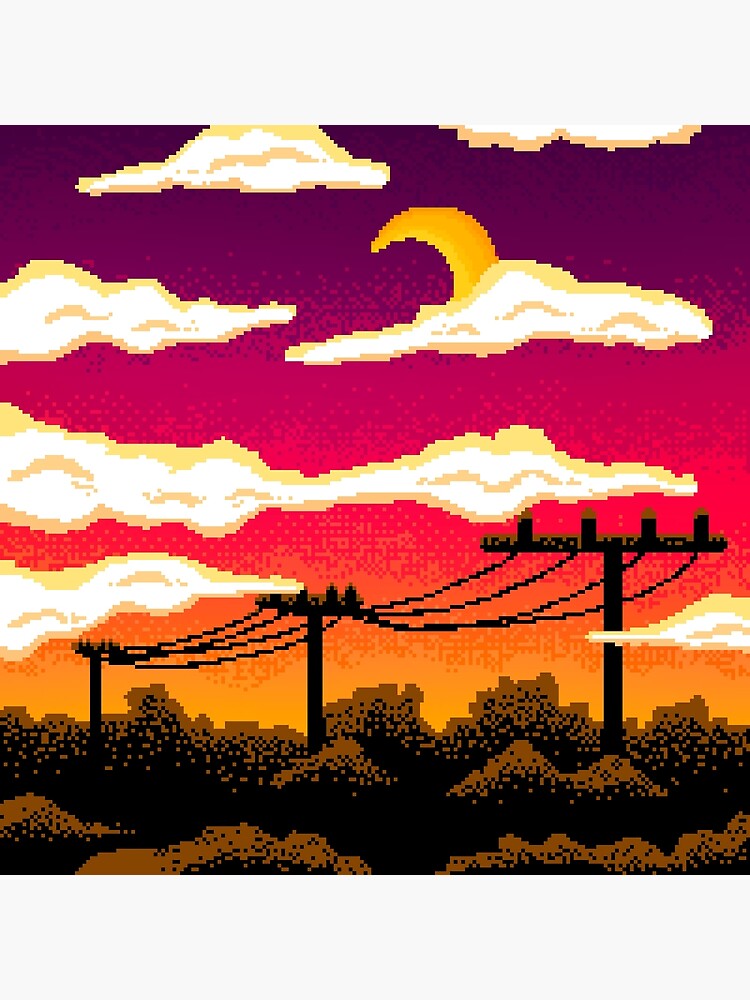This vibrant drawing, reminiscent of retro 2D pixelated art, depicts a sunset scene with three telephone poles connected by wires, stretching diagonally from the left to the right. The sky transitions seamlessly from yellow at the horizon, through orange, pink, and maroon, to deep purple at the top, with golden-bordered clouds scattered throughout. Nestled among the clouds, a golden crescent moon shines brightly. Below, the dark brown and black-shadowed treetops, appearing pixelated, blend into the bottom of the image, creating an abstract, shadowy foreground that suggests the silhouettes of bushes or trees against the radiant sunset sky. The image evokes a nostalgic feel, akin to a classic 8-bit video game, and could easily serve as a striking piece of art in a home.